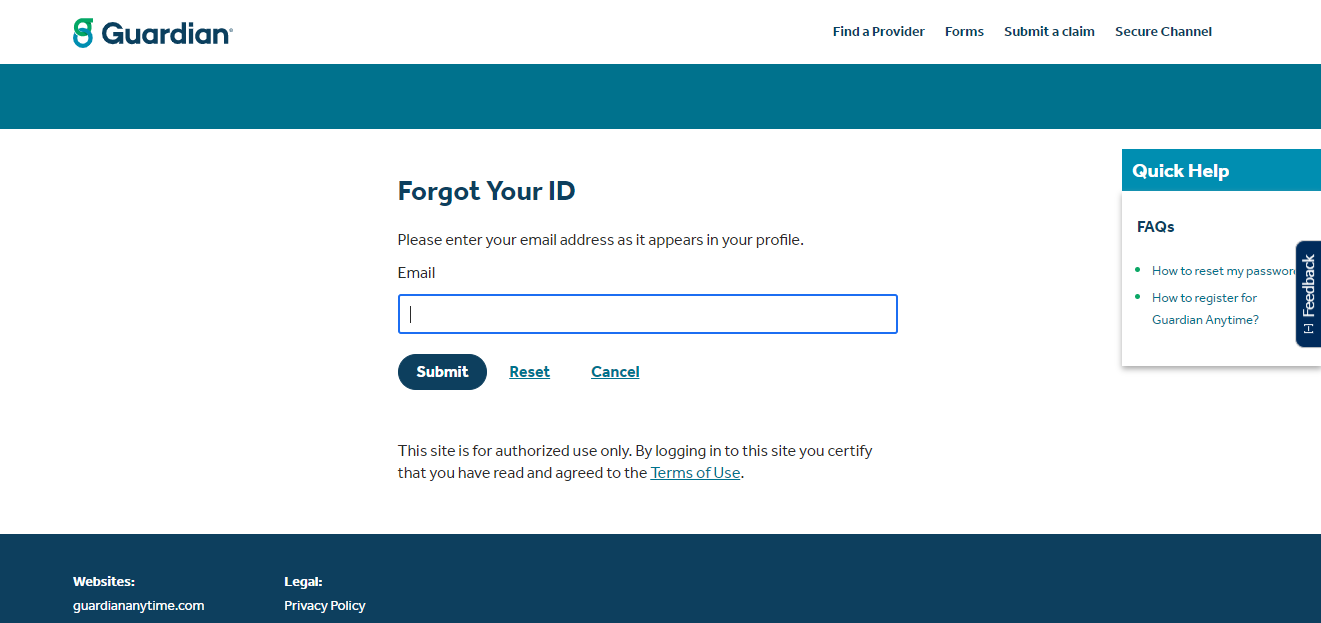This screenshot displays a webpage from a user’s computer, specifically a login assistance page for a service called "Guardian." 

In the top left corner of the interface, "Guardian" is prominently displayed in black text. Situated to its right are a series of navigation options, including "Find a Provider," "Forms," "Submit a Claim," and "Secure Channel."

A dark blue, almost teal, border encompasses the page, framing a central white section that is designed to help users recover their account IDs. In this white area, the header "Forgot Your ID?" is printed in black, followed by the prompt, "Please enter your email address as it appears in your profile." Below this text is a field labeled "Email," accompanied by a blue input bar.

Further down, three buttons are lined up horizontally: "Submit," "Reset," and "Cancel." Beneath these buttons, a security reminder states, "This site is for authorized use only. By logging into the site, you certify that you have read and agreed to the terms of use," with "terms of use" highlighted in blue, indicating it is a clickable link.

On the right side of the page, there is a "Quick Help" box featuring a list of useful topics such as "Facts," "How to Reset My Password," and "How to Register for Guardian Anytime."

At the bottom of the screen, a slightly darker blue strip contains the website's address, "GuardianAnytime.com," and a link to the legal privacy policy.